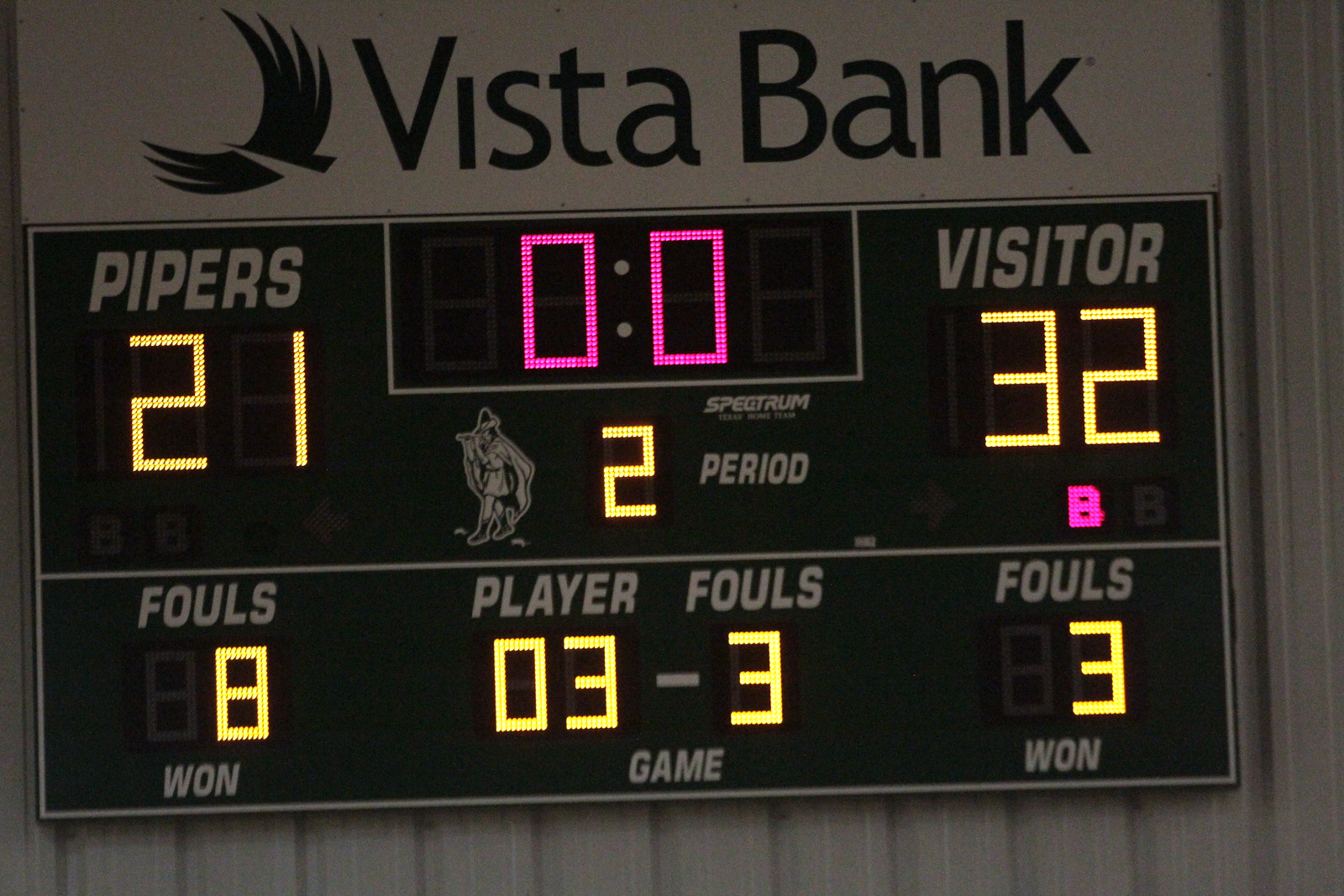The image depicts a mostly black and white scoreboard sponsored by Vista Bank, prominently displaying the bank's name in white letters along with a drawing of a bird. The scoreboard is situated on a gray or silver aluminum siding, indicating a modern, indoor setting, likely a gymnasium. The top part of the scoreboard shows "Pipers," who have a score of 21, and "Visitor," with a score of 32, in yellow numbers. It also indicates that it is the second period of the game with both teams having varying fouls. The Pipers have accrued eight fouls while the Visitors have only three. Notably, player three has three fouls, though it is unclear which team they belong to. The timer displayed in pink reads 0-0, possibly indicating the end of the game. The Vista Bank logo and names are slightly off-center towards the top of the image, and the color scheme consists of white, black, yellow, and some pink for the timer. The wall behind the scoreboard, possibly aluminum siding, is a darkened gray or silver, contributing to the scoreboard's prominent display.